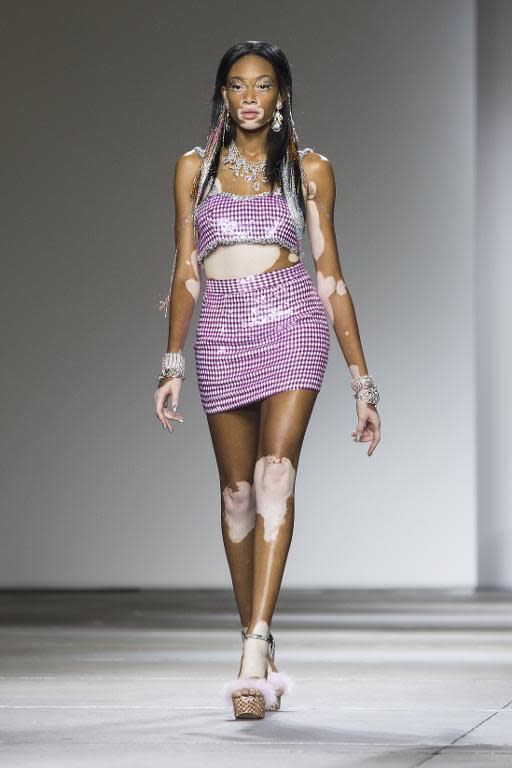The image features a model confidently walking down a white runway. She exhibits a skin condition called vitiligo, characterized by lighter patches around her mouth, fingers, knees, ankles, belly, and elbows, contrasted against her otherwise dark skin. The model dons a striking ensemble: a sleeveless, purple checked crop top paired with a matching short skirt. Her attire is accentuated with shiny silver details, and she accessorizes with a prominent silver collar, large silver earrings, thick silver bracelets, and a necklace embellished with diamond-like studs. Her nails are painted a metallic silver, and she wears eye-catching high heels adorned with pink fluff. Completing her sophisticated look, she has long black hair and wears makeup with pink lipstick and silver eyeshadow. The all-white backdrop of the runway and its floor complement her stunning appearance.